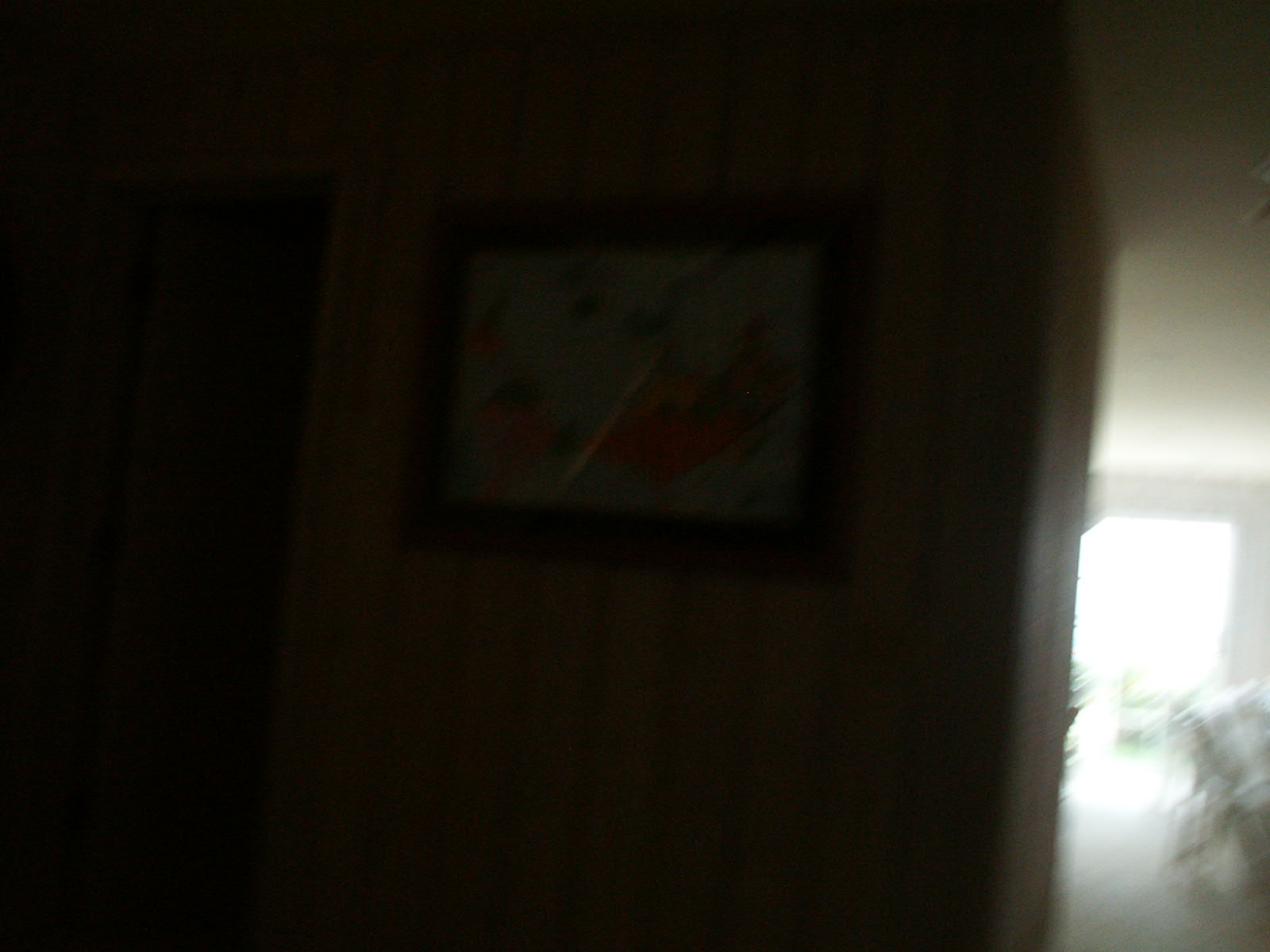This is a dark and blurry photograph of the interior of a house. The image, which is slightly wider than it is tall, prominently features a tan-colored wall with vertical brown divisions. Hanging centrally on the wall is an almost rectangular, square-shaped frame with a dark border—it appears to be a clock, though its face is indistinct due to the darkness, showing only a single gold hand clearly. Above the clock is another frame, possibly a picture, characterized by a brown border with a teal interior, depicting pink flowers surrounded by green, leaf-like shapes. To the right of this wall, about 20% in from the edge, is a doorway leading to a well-lit room illuminated by sunlight streaming through a window. On the left, there is a completely darkened doorway, adding to the overall dimness of the scene. There is also a green object, likely a plant, hanging on the darker part of the wall. The photograph captures no people or text.